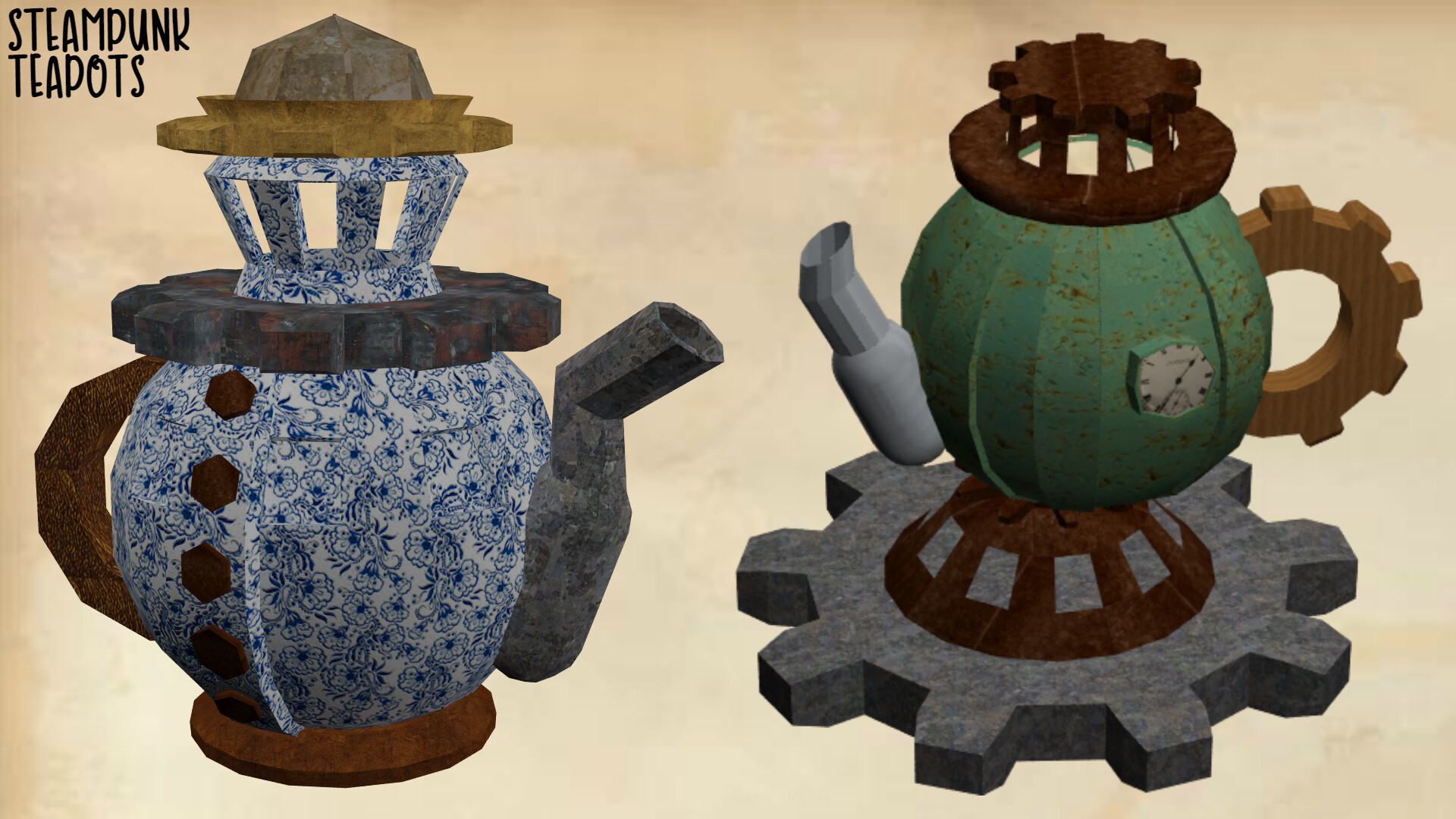In a computer-generated image labeled "Steampunk Teapots" at the top left, two intricately designed teapots are prominently displayed against a neutral brown and white backdrop. 

The teapot on the left side is blue and white, adorned with tiny swirling blue designs. Its spout appears dark gray, and it features four brown buttons, giving it a whimsical, almost anthropomorphic appearance. Its neck and "hat" are reminiscent of metal gears, and it sits atop a copper base, enhancing its steampunk aesthetic. The overall texture suggests a blend of stone and artificial craftsmanship.

On the right side, the green teapot has a solid, slightly rusted appearance and is more overtly mechanical. It too incorporates a large metal gear into its design. The handle is yellow, while the spout is light gray. This teapot rests on a mechanical wheel, further emphasizing its industrial and machine-like character.

Both teapots, sharing a steampunk theme, exude an industrial yet fantastical charm, combining elements of Victorian-era design with mechanical intricacies, making them appear almost lifelike yet distinctly artificial.